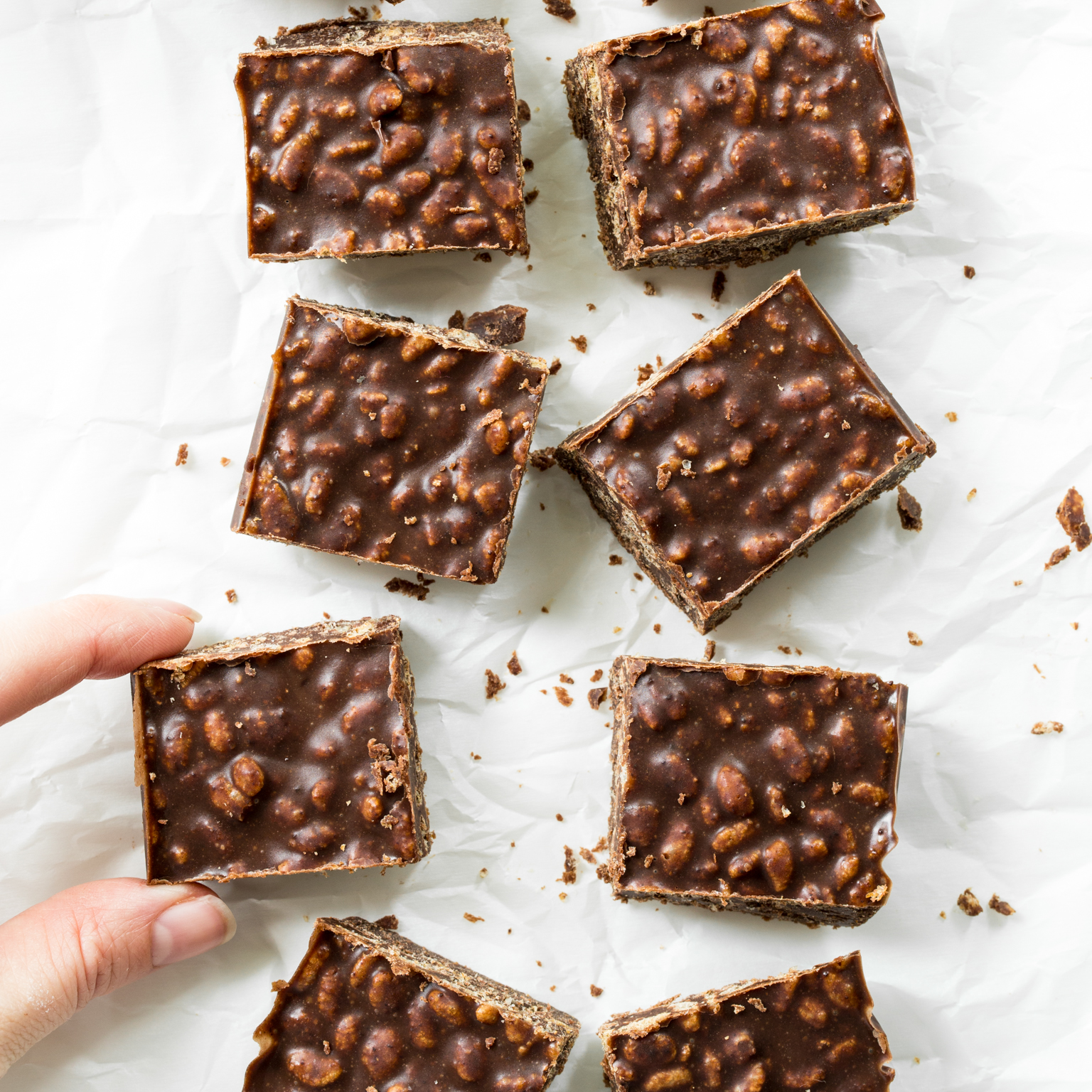A close-up color photograph showcases eight homemade squares of rich, dark brown chocolate fudge, adorned with nuts that are both embedded within and sprinkled atop the treats. These fudge squares are cut in a two-by-four arrangement, with each piece roughly measuring two inches by one and a half inches. The pieces are set against a pristine white, slightly marbled surface, giving a clean, bright backdrop that contrasts with the dark fudge. To the left, a Caucasian hand emerges, with the fingers delicately pinching one piece of the fudge, poised to lift it. The hand is clearly visible showing the index finger and thumb grasping the treat. The fudge appears slightly crumbly, with small flakes scattered around, enhancing the homemade, rustic appeal. The overall color palette of the image includes rich dark browns, lighter beige tones of the nuts, the white of the countertop, and the flesh tones of the hand.